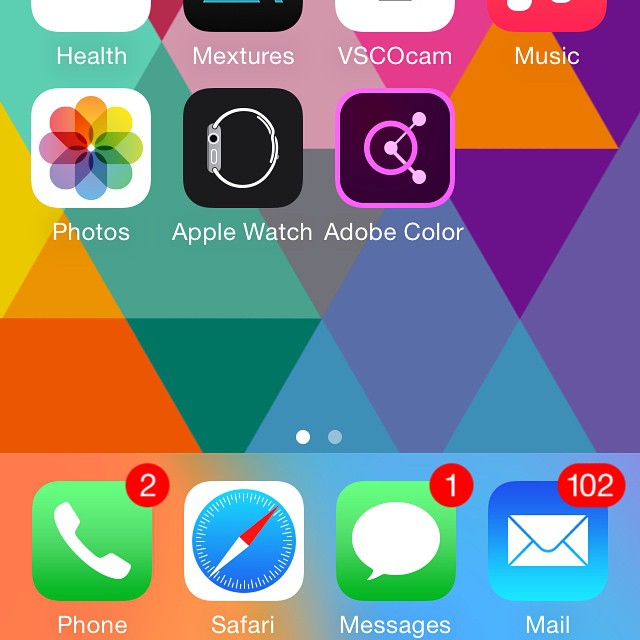A close-up shot of an iPhone's bottom half of the home screen reveals a detailed view of the user's application layout and notifications. The dock at the bottom of the screen features four quick shortcut icons: Phone, Safari, Messages, and Mail. Above the dock, half of four icons from the first home screen row are visible: Health, Mixtures, VSCO, and OCam, while in the next row, the full icons for Photos, Apple Watch, and Adobe Color are present. The background displays a vibrant geometric pattern composed of triangles in various colors and shades, including orange, yellow, green, gray, purple, and pink. Notification indicators show two missed calls on the Phone icon, one unread message in the Messages app, and a significant 102 unread emails in the Mail app.